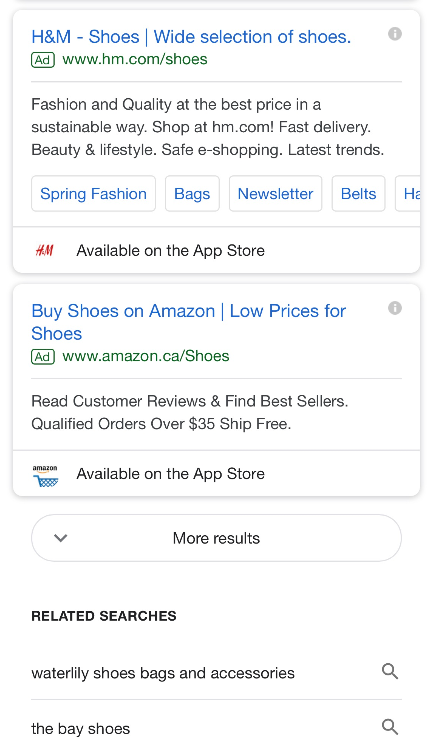A screenshot of Google search results for "shoes" taken on an iPhone, displaying two advertisements at the top. The first ad is from H&M, showcasing a wide selection of shoes, while the second ad promotes buying shoes at low prices on Amazon. Both ads indicate their availability on their respective apps via the App Store. The search results page has a button labeled "More results," suggesting further exploration is possible. Below the ads, a section titled "Related searches" includes terms like "water lily," "shoes, bags, and accessories," and "the bay shoes," indicating recent activity. Additional sub-links under the H&M ad offer quick navigation to specific categories such as spring fashion, bags, newsletters, and belts. The page features a clean layout with predominantly white background, black text, and green highlights for advertisements.